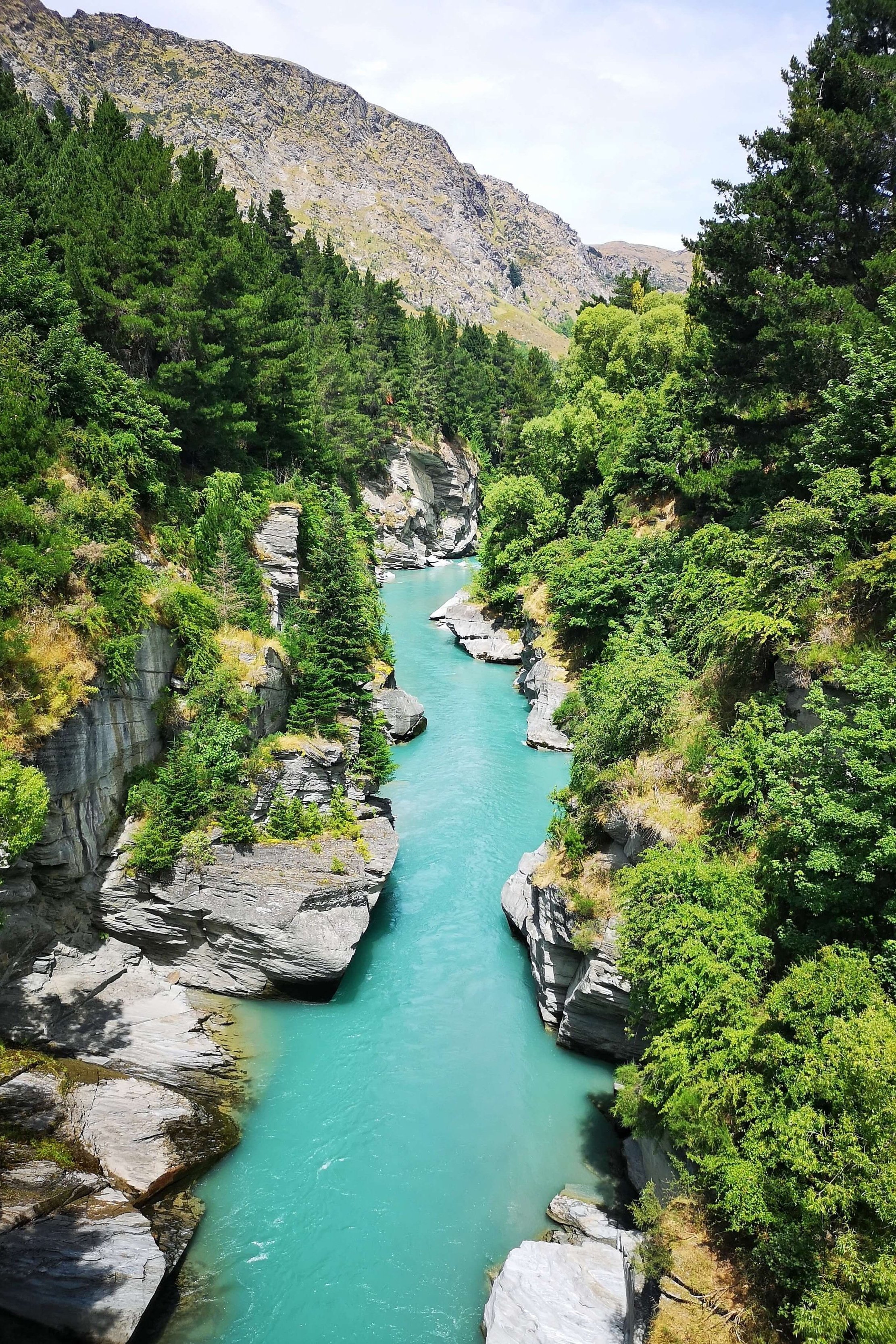This vertical, slightly cyan-tinted photograph captures a scenic aerial view of a serene and untouched wilderness, centered around a crystal-clear, turquoise-blue river. The river flows through a narrow, rocky gorge, its banks lined with large, gray boulders and sharp cliff-like edges that drop steeply into the water. In the foreground, dense clusters of tall, green evergreen and pine trees thrive, some even growing bravely from the rocky banks right along the river. Moss patches can be glimpsed on rocks partially submerged in the water. The gorge is enveloped by a forest, adding to the lush greenery, while in the background, a bare, rocky mountain devoid of vegetation stands tall under a sky dotted with clouds. This photograph exudes a peaceful and tranquil ambiance, devoid of human presence, boats, or animals, making it an alluring snapshot of pristine natural beauty.